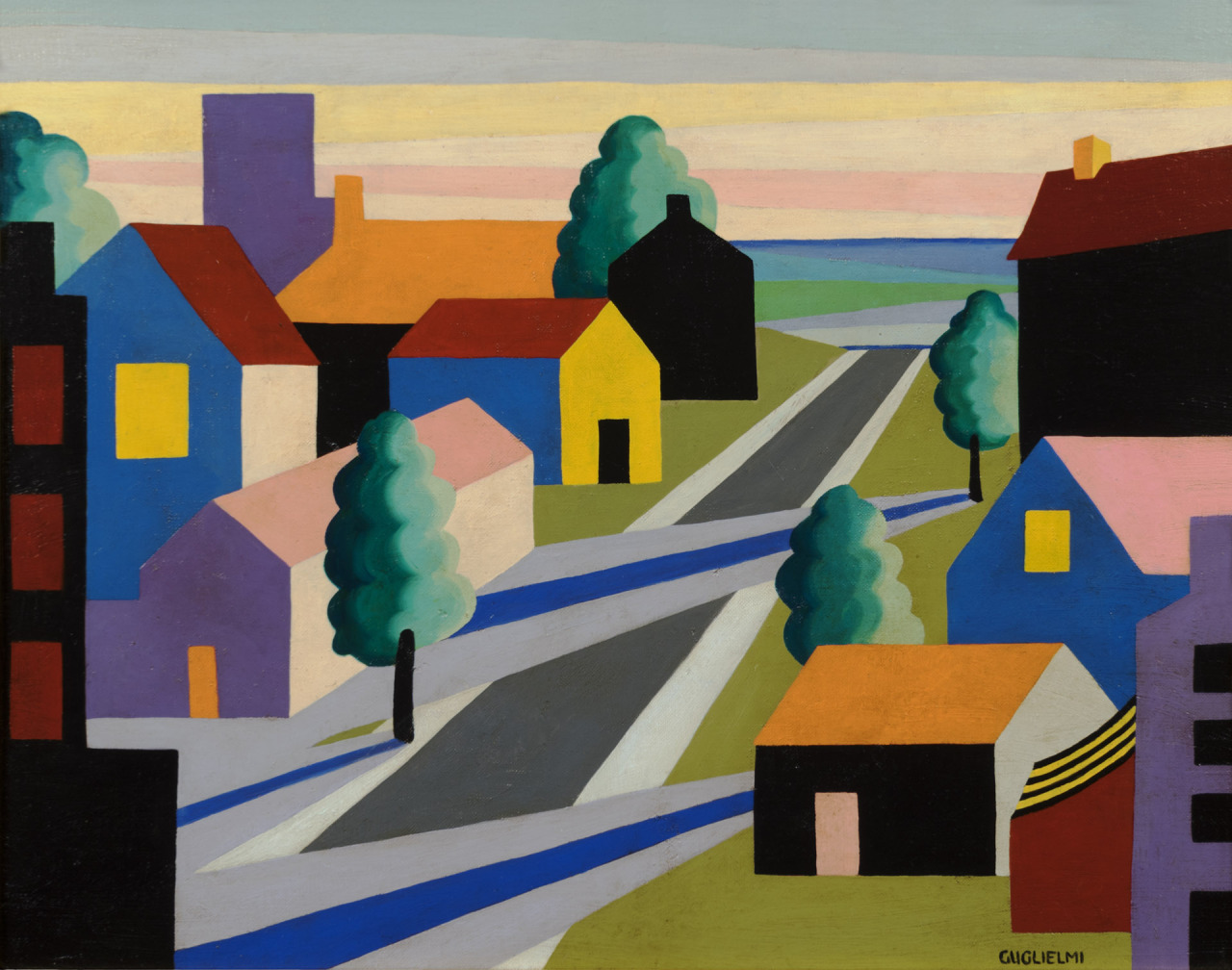The image is a vibrant and abstract painting of a small town or village, prominently using structured shapes and a multitude of colors. The sky is divided into horizontal strips of various colors, starting with blue, followed by light blue, yellow, beige, peach, and ending with another beige strip. Beneath the sky, an abstract sea and stretch of green likely represent water and grass. 

In the foreground, a long gray road runs vertically, intersected by two horizontal gray strips marked with a blue stripe. On either side of this road, there are colorful buildings and trees. The buildings are painted in block colors: some have red roofs with blue, yellow, or white walls, and doors and windows in contrasting hues like black and yellow. One building is pink, violet, and beige, while another features a blue side, a red side, and a yellow side.

The landscape includes green puffy-leaved trees with black trunks positioned strategically on both the left and right sides of the road. The artistic style is characterized by a use of bold colors and abstract forms, providing a lively and dynamic representation of the small town setting.